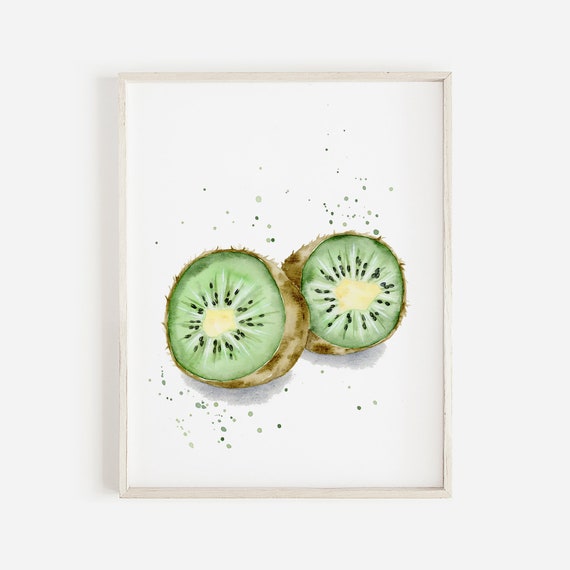The image depicts a detailed painting prominently featuring two halved kiwis, serving as the central focus of the artwork. Both kiwis are aligned slightly offset, with the one on the left positioned a bit lower than the one on the right. They reveal vibrant green interiors accentuated by yellowish-white cores surrounded by delicate black seeds, all encased in a tannish-brown outer layer. The kiwis are depicted as though splattered with small specks of green paint both above and below them, adding dynamic details to the otherwise pristine white background. This artwork, showcased in a clean white frame against a stark white wall, emphasizes the natural beauty and simplicity of the kiwis, set against a minimalist backdrop that draws the eye directly to the central fruit figures.